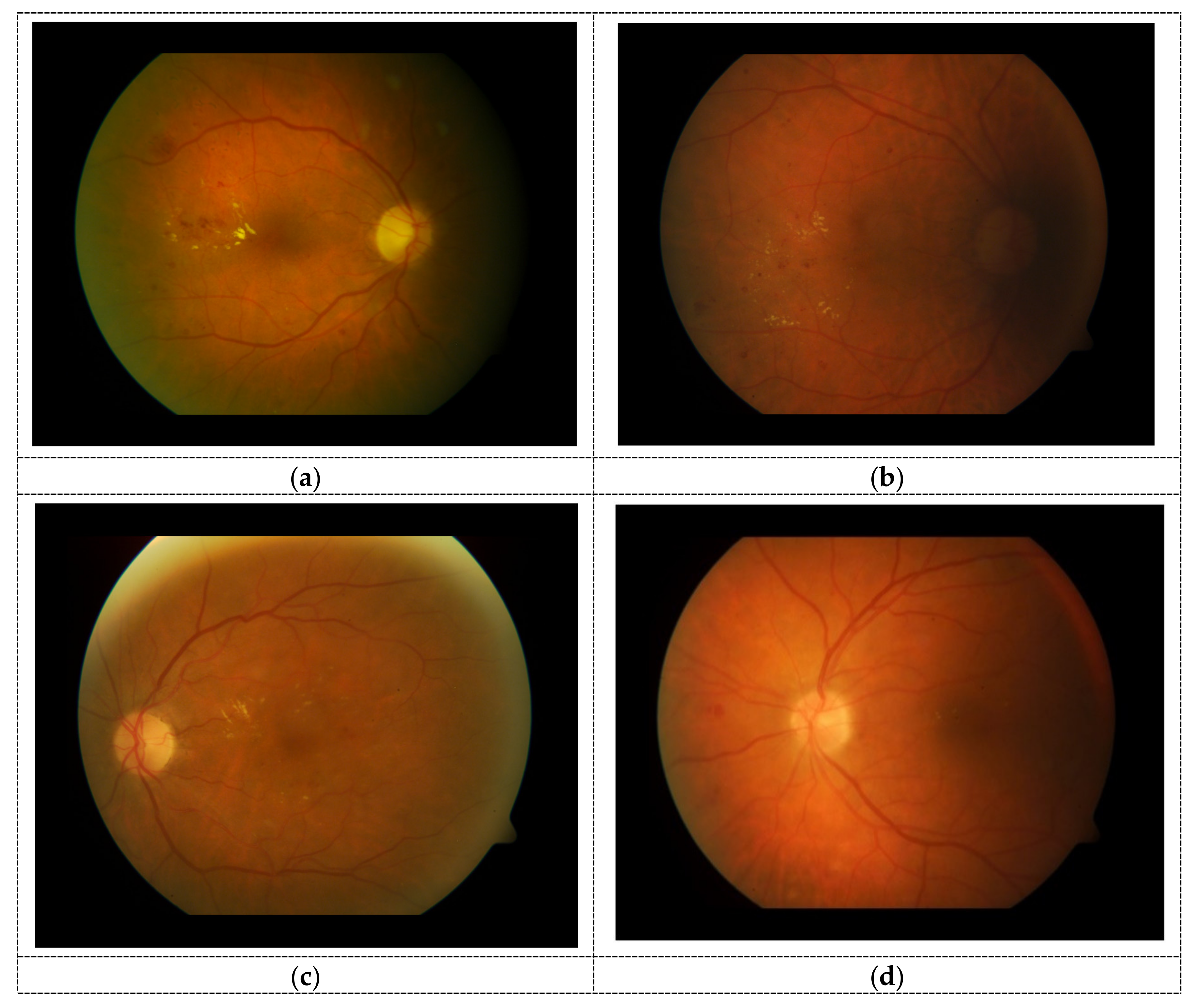This is a collection of four photographs, likely from a scientific publication, showcasing biological tissue. Each image is circular and displayed against a black background, organized in a grid with labels A, B, C, and D in parentheses. 

In image (A) at the top left, the tissue features a bright yellow dot located at the center-right, set against a reddish veined backdrop. Image (B), found at the top right, shows a darker version of this tissue where the yellow dot has disappeared, leaving the reddish veins more prominent in the dimmer setting.

Moving to the bottom row, image (C) on the lower left presents the yellow dot now positioned on the left side of the tissue, yet the red veins retain their placement. Lastly, image (D) at the bottom right shows the yellow dot transformed to a more muted orange hue while the red veins remain consistent across all images.

Overall, despite the varying placements and visibility of the yellow dot, the reddish veins hold a steady presence throughout the series, providing a detailed and potentially insightful look at the changes perceived in the biological sample.